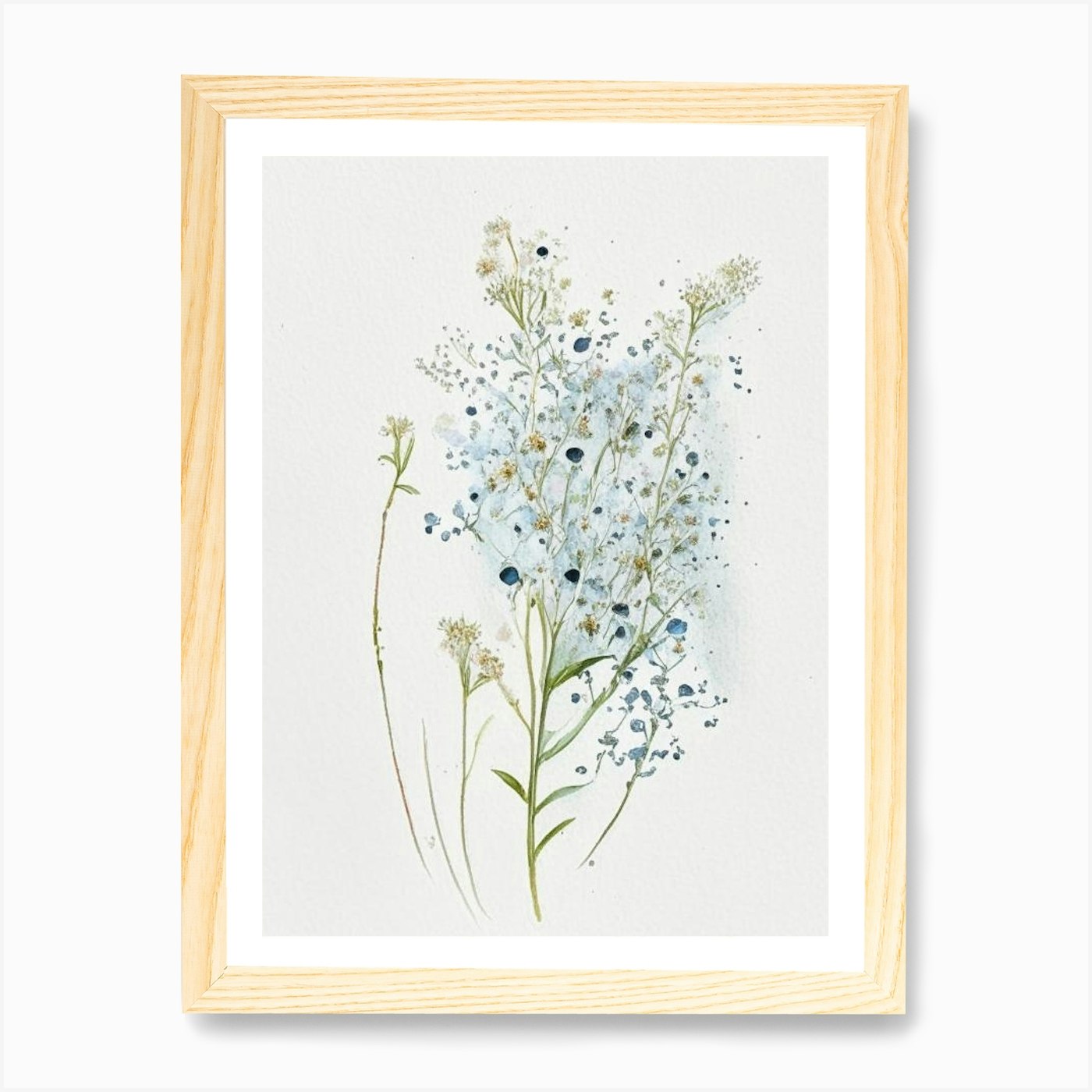This image features a detailed painting of blue flowers with smatterings of yellow and green accenting the petals and leaves. The flowers, which are attached to green stems with some light brown hues, stand out against a subtle light blue background. Interspersed among the flowers, there are various sizes of darker blue dots, some large and some small. The painting is bordered with a white mat, which itself is surrounded by a light brown wooden frame that has darker brown lines and grooves. The corners of the frame have a slightly whitewashed appearance. The entire composition is set against an all-white backdrop, further emphasized by the soft gray shadows at the bottom and right side of the image.